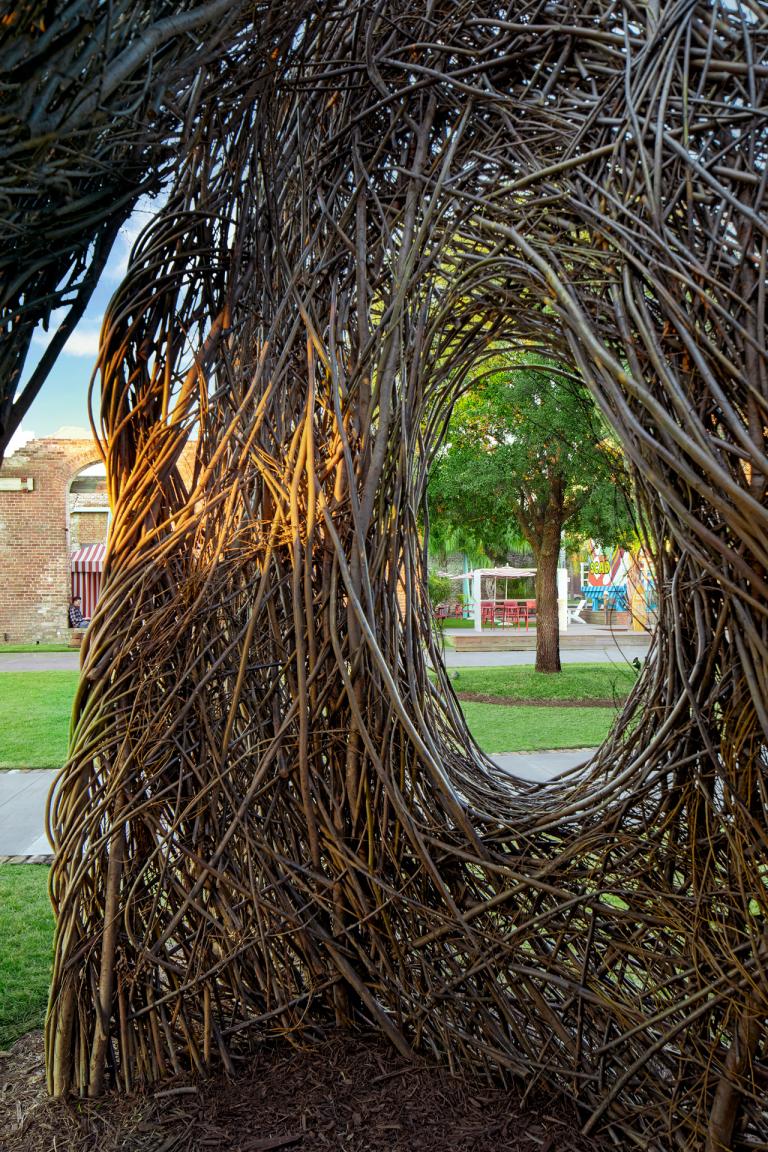The image showcases a detailed and artfully crafted sculpture made of roots or vines, intricately woven into a large, vertical, donut-like shape. This natural sculpture frames a prominent circular opening in the center. Through this framed circle, one can see a tree sprouting from a well-maintained lawn, set against a backdrop of buildings that resemble restaurants or coffee shops. There's also a walking path enclosed within the green surroundings, indicating that this scene is set in a park or plaza. Additionally, the photograph captures clear skies above, suggesting a bright, sunny day. The perspective of the image, taken during daylight, adds to the vibrancy of the scene, with the natural sculpture and its surroundings basked in shadow of larger trees, or structures nearby. Both the artistry of the woven roots and the serene, urban environment create a strikingly picturesque and tranquil setting.